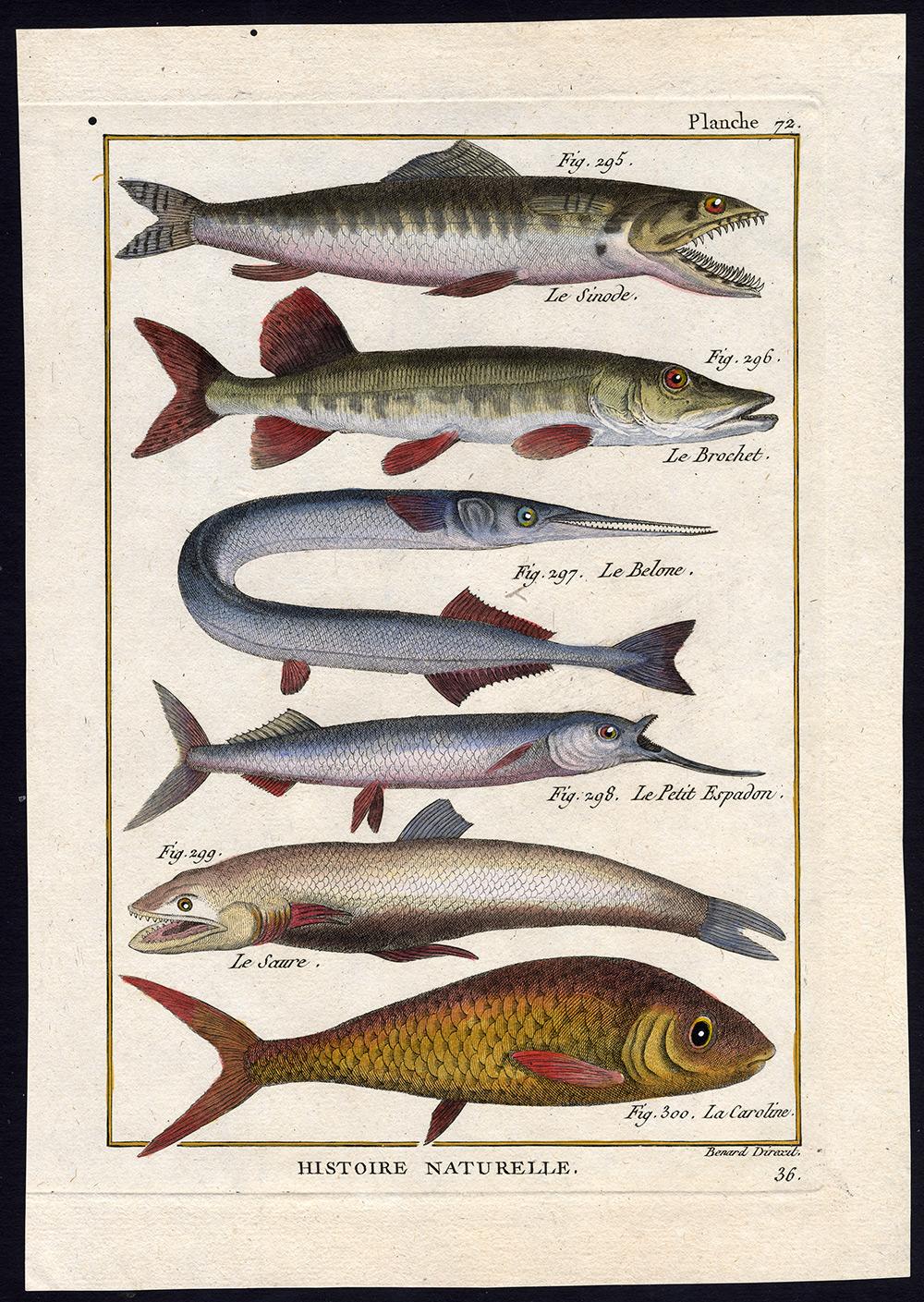This detailed vintage print, framed with a black border and white matting, showcases a series of ancient fish illustrations. At the top, the print is labeled "Planche 72" with various numbered figures. The first figure, "Figure 295," depicts "Le Senod," a green and white fish characterized by its razor-sharp teeth. Below it is "Le Brochet" (Figure 296), a long fish with green and white scales.

Further down is "Le Bellone" (Figure 297), a long, gar-like fish depicted in a curved, almost eel-like form. Following this is "Le Petit Espadon" (Figure 298), distinguished by a prominent, elongated lower jaw. Next, "Le Saure" (Figure 299) features a stocky body with short, sharp teeth. The final image at the bottom is "La Caroline" (Figure 300), showcasing a fish with a high arched backbone and distinct red fins. 

All fish are oriented with their heads pointing to the right, except for the one in "Figure 299" which faces left. The bottom of the print is marked "Histoire Naturelle, 36." This historically rich illustration not only identifies each fish but also hints at their potentially scientifical or regional significance.